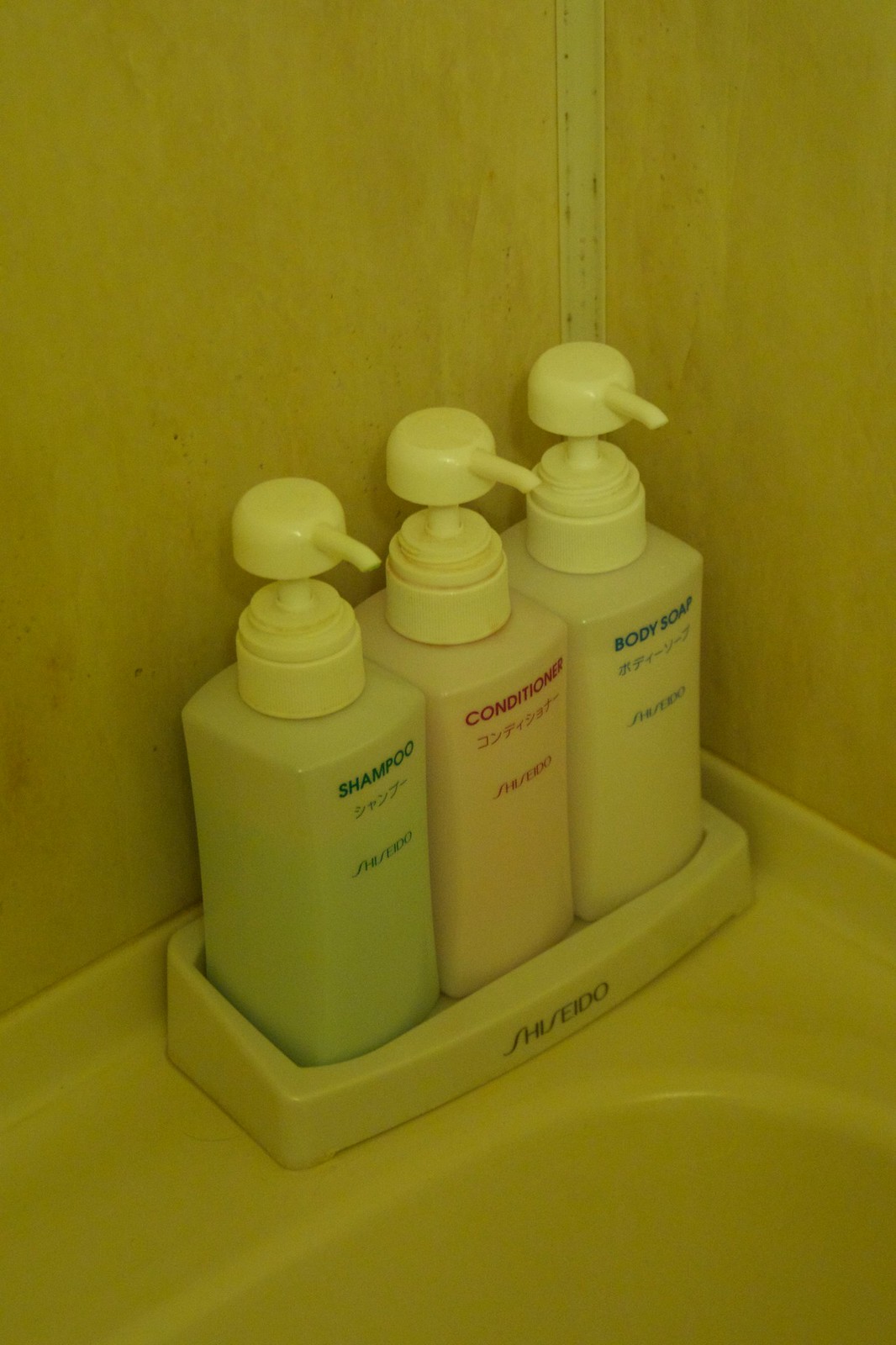This photograph captures a close-up view of the corner of a bathtub inside a bathroom. Resting on the edge of the porcelain tub, which is tinged yellow likely due to the lighting, is a sleek plastic base holding three uniform pump bottles. The base, branded with the Shiseido logo, is designed to fit these three containers perfectly. Each bottle features a flat white pump with a thin nozzle. The bottles contain different products, as marked by their labels and corresponding colors: the left bottle, tinted blue, is labeled "Shampoo" with Japanese characters underneath; the middle bottle, tinted pink, is labeled "Conditioner," also accompanied by Japanese characters; and the right bottle, containing a white liquid, is labeled "Body Soap" with similar Japanese text. The overall composition and consistent branding suggest a cohesive and organized arrangement of high-quality Japanese bath products.